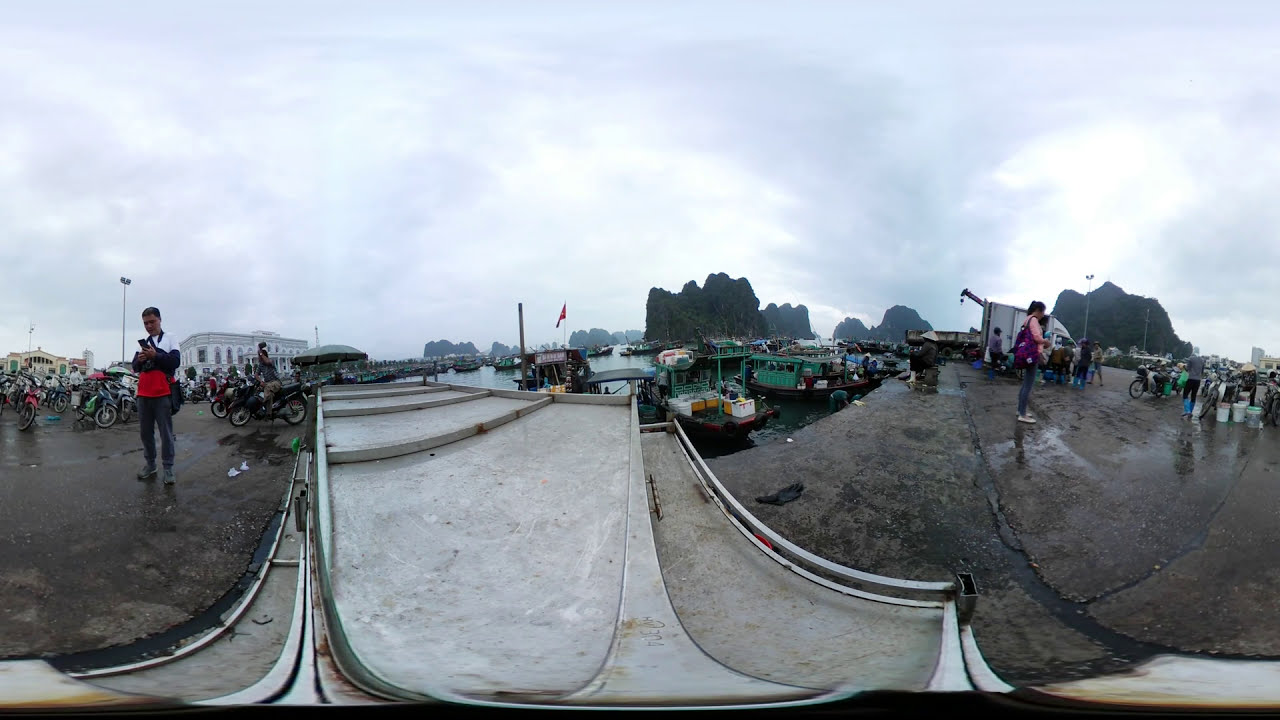In this horizontally aligned rectangular picture, the top half is dominated by an overcast sky, blending shades of white and gray clouds, indicative of recent rain. The large paved area below appears dark gray and wet, with puddles scattered around. In the middle of the image lies a peculiar feature that resembles a gray roadway with some steps, bordered by brownish-gray worn walkways.

On the left side of the image, a darker-skinned man dressed in a white, black, and red long-sleeved shirt can be seen. He has short, dark hair, jeans, and dark-colored shoes, holding a dark object—perhaps a phone—in front of him. Behind him, a long row of motorcycles lined up against a large white building catches the eye. A man sits on one of the bikes, adding to the bustling activity, along with people walking around.

To the right, a woman with a black ponytail wearing a long-sleeved pink shirt, jeans, and white sneakers examines something in her hand. She wears a purple backpack, adding a splash of color to the scene. More motorcycles are visible in the background behind her. Additionally, to her left, there is a small water body with several boats tied up at the docks and trees in the background. The overall scene is framed by distant rocky cliffs, enhancing the sense of a moody, rainy day.